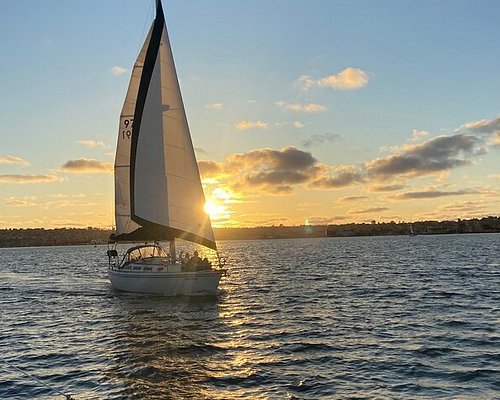A pristine white sailboat glides smoothly over the still, crystal-clear blue waters of the ocean, its sails fully raised and catching the light breeze. The serene scene is bathed in the warm, golden hues of an impending sunset, with the sun hovering just above a barely discernible landline that stretches across the horizon from left to right. The sky overhead is a mix of light and dark clouds, adding depth to the tranquil summer evening ambiance. On closer inspection, two or three figures can be seen aboard the sailboat, positioned towards the front and rear, enjoying their peaceful journey towards the distant, indistinct coastline, which may host some houses and lush forests. The tranquil waters reflect the soft light of the setting sun, adding a shimmering effect to this idyllic maritime scene. The absence of other boats or marine life only emphasizes the calm and undisturbed nature of this picturesque moment.